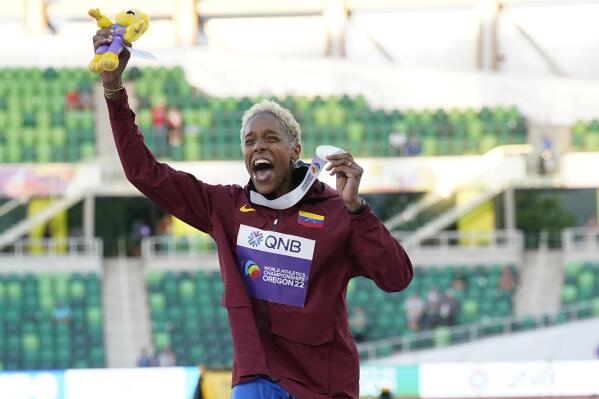In the image, we see a jubilant athlete, a black woman with blonde hair, celebrating her triumphant finish. She is holding a silver medal in her left hand, lifting it proudly beside her face. In her right hand, she holds a small, yellow stuffed toy adorned in purple clothing. The woman is dressed in a maroon or burgundy overcoat, which features a square emblem on her chest with the top half white, bearing the text 'QNB,' and the bottom half purple. Positioned against a blurred backdrop of sparsely filled green seats in a sports arena, it’s evident she has won a race or some type of sporting event. Her exuberant expression exudes happiness and pride, symbolizing her great achievement at what appears to be an event marked with "Oregon 22."